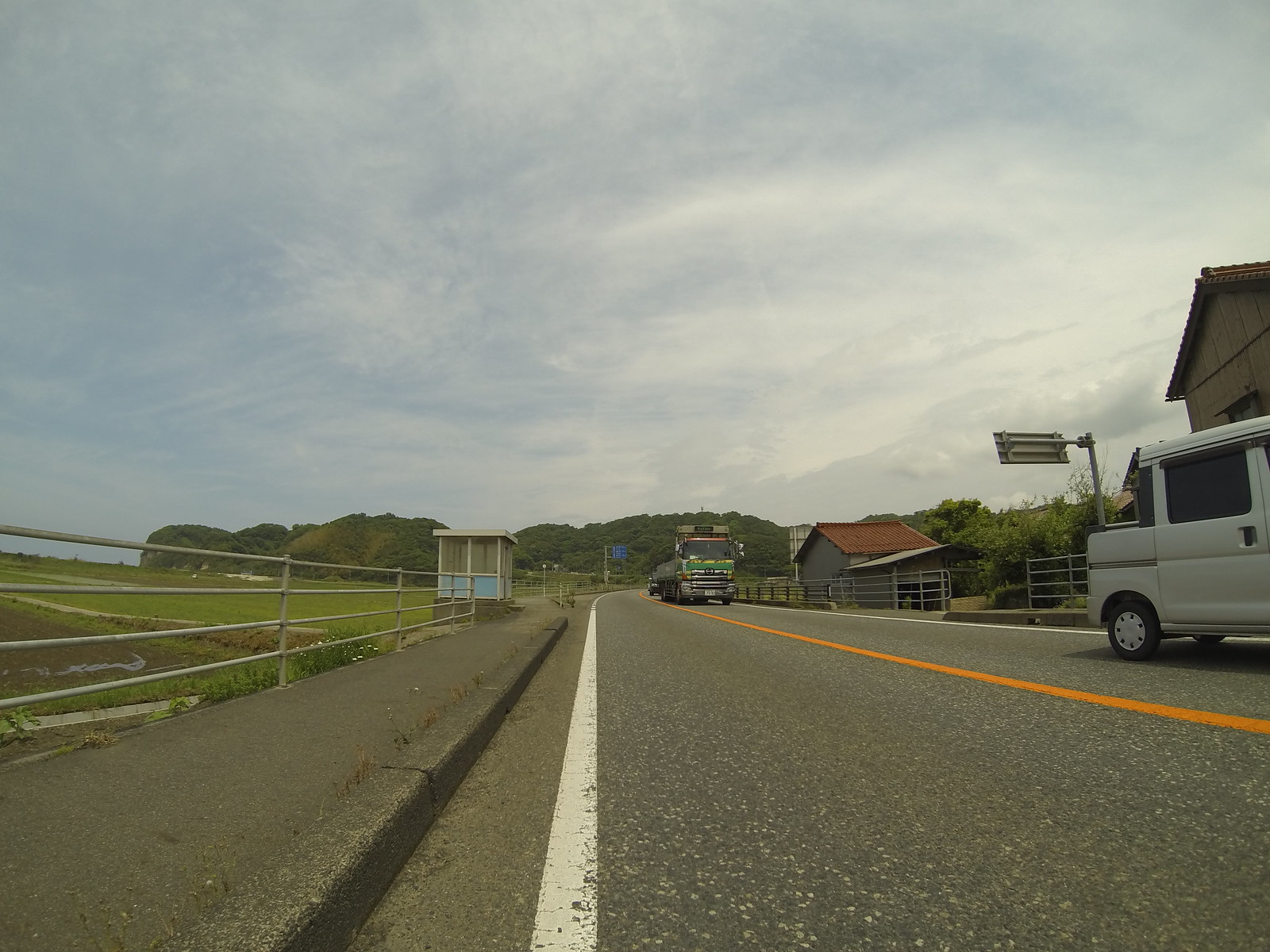The image captures a two-lane road with a white line running close to the camera along the road's left edge, aligned with the solid yellow median line. On the right side of the road, a white van is moving, while in the distance, a green tractor-trailer appears to be heading towards the camera but positioned on the left, hinting at vehicles either being parked or traveling in opposite directions. Flanking the road are metal guardrails, and to the left, beyond a narrow concrete barrier and four-railed metal fence, lies an expansive grassy field. This field extends to a distance where rows of tall trees frame the horizon. On the right side, near the midpoint of the image, a small wooden shack is visible with additional single-story wooden buildings peeking just above the van. The scene is set against a partially cloudy blue sky, adding a serene backdrop to the bustling road.